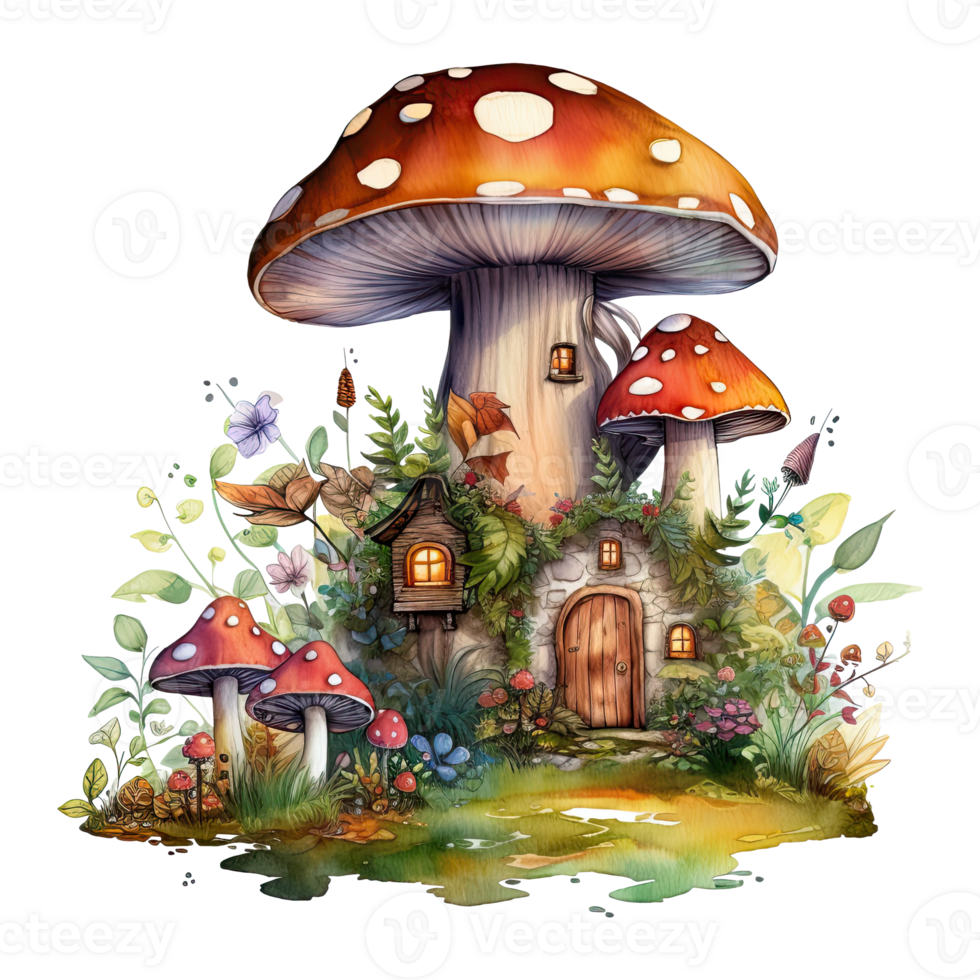The illustration is a charming, fantastical scene depicting a small house nestled at the base of an enormous, iconic red-capped mushroom adorned with white spots. This main mushroom, which looms protectively over the structure, features a light beige and white underside and stem. The house itself has a wooden brown door at its base, flanked by several small windows radiating a warm, golden glow, suggesting a cozy interior. Surrounding the house, a variety of smaller mushrooms, differing in shapes and sizes, intermingle with colorful flowers and lush flora, creating a vibrant, whimsical environment. The watercolor-esque artwork showcases detailed plant life, including grass, flowers, and vines, adding to the enchanting and serene atmosphere of this fantasy setting. The entire composition gradually fades out at the bottom, enhancing its dreamlike quality.